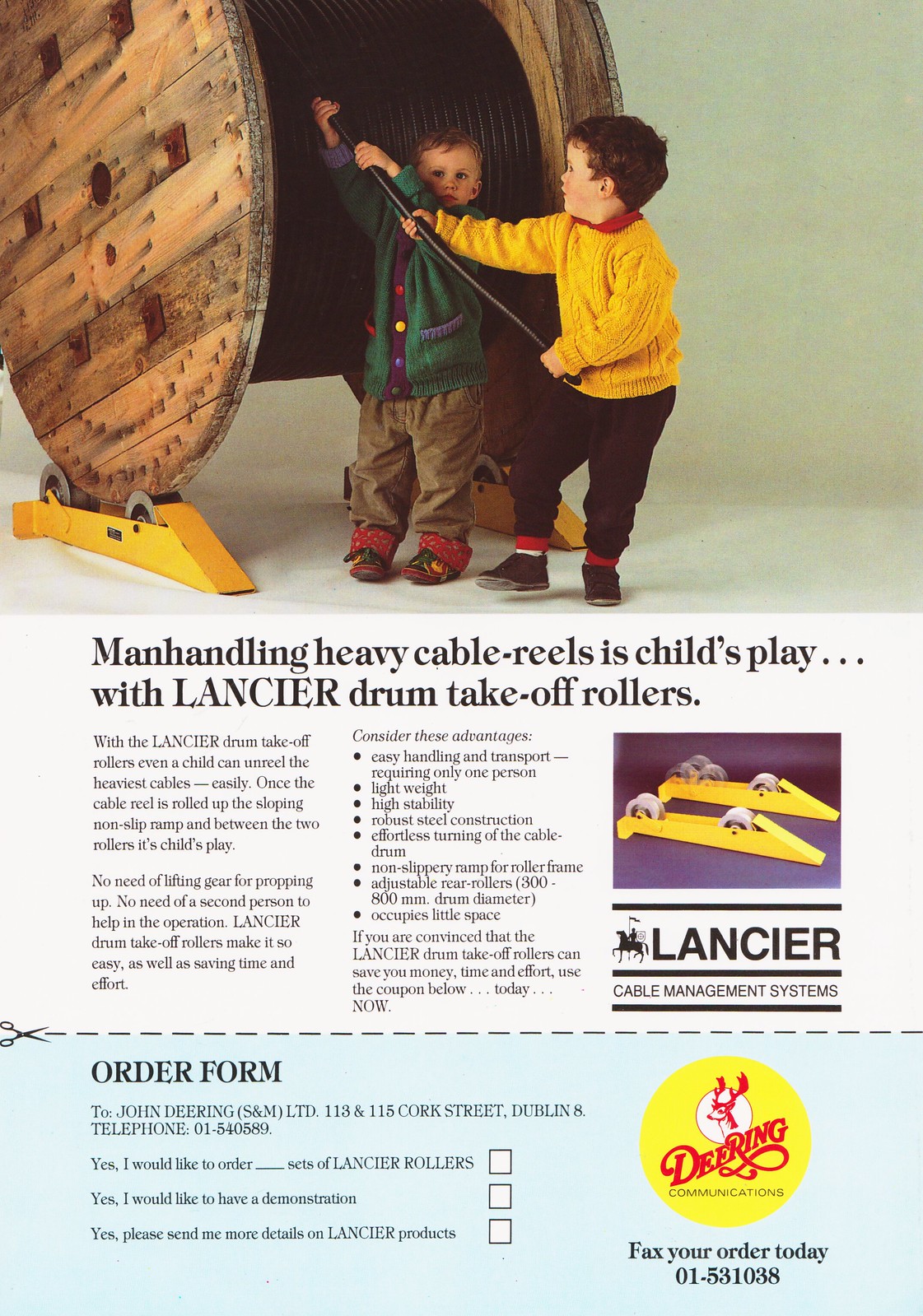In this advertisement for Lancer drum take-off rollers, the focal image at the top shows two young children easily pulling a black cable from a large wooden cable reel stabilized on two yellow, sloping, non-slip platforms. The child on the left, wearing a green jacket, purple sweater, brown trousers, and shiny sneakers, looks directly at the camera, while the child on the right, dressed in a yellow sweater with red collars, black trousers with red borders, and black sneakers, focuses on pulling the cable. Accompanying this image is text emphasizing the product's ease of use: "Manhandling heavy cable reels is child's play. With Lancer drum take-off rollers, even a child can unreel the heaviest cables easily. Once the cable reel is rolled up to the sloping, non-slip ramp and between the two rollers, it's child's play. No need for lifting gear or a second person. Lancer drum take-off rollers save time and effort."

To the right of the main image, there's a detailed picture of the yellow ramp and rollers. Beneath the images, text elaborates on the product’s advantages: "easy handling and transport requiring only one person, lightweight, high stability, robust steel construction, effortless turning of the cable drum, non-slippery ramp for roller frame, adjustable rear rollers for 300-800 mm drum diameter, and minimal space occupation."

At the bottom, there's a blue-background order form bordered with a scissor icon for cutting out. The form, decorated with the Lancer brand logo featuring a black horse and a rider holding a flag, and another logo reading "Deering Communications" in yellow with a deer image, prompts potential buyers to fax their orders to John Deering at S&M Limited, 113-115 Cox Street, Dublin 8. The form includes options to order sets of Lancer rollers, request a demonstration, or ask for more details, followed by the contact number, 01531038.